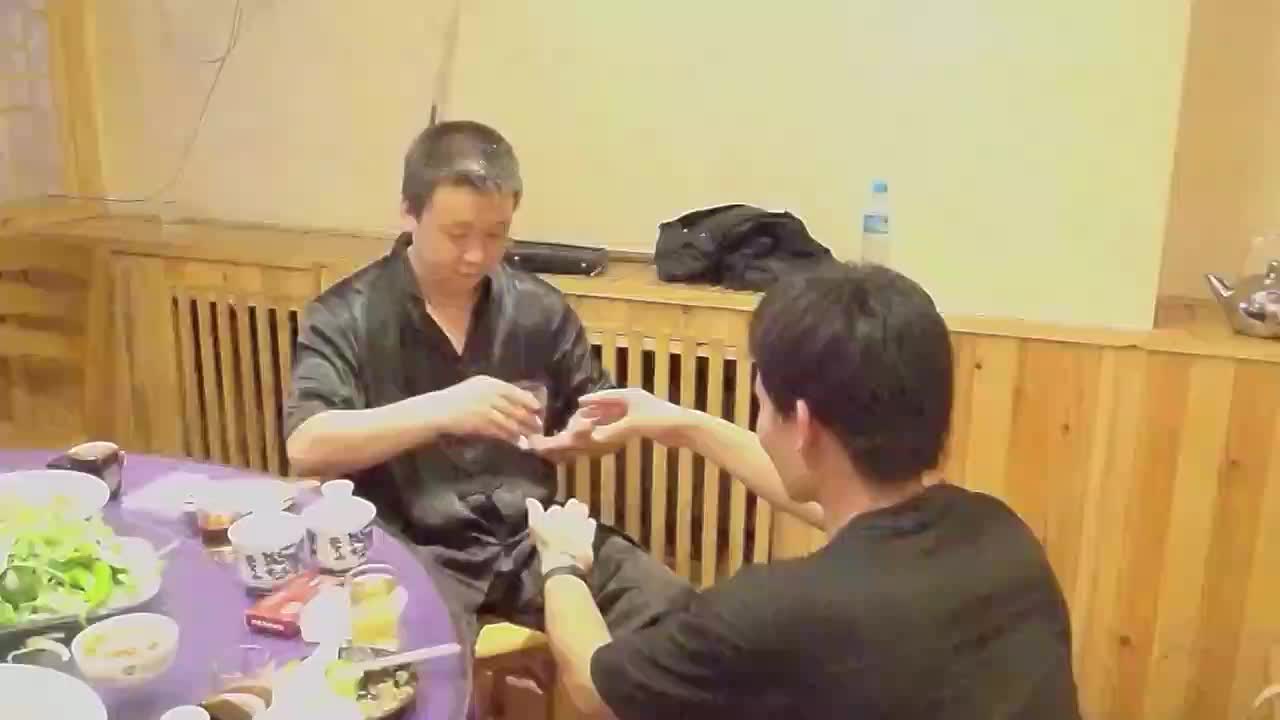In a warmly lit restaurant with beige walls and wooden wallpaper accents, two Asian men are seated at a round table covered with a purple tablecloth, laden with a sumptuous spread of Chinese food. The man on the left, dressed in a black button-down shirt and pants, faces the camera with his eyes closed while holding a clear glass of liquid. His companion, wearing a black t-shirt and with short black hair, faces away but reaches out with both hands, eagerly anticipating the drink. The table is filled with bowls of tea, vibrant green bok choy, cabbage dishes, and numerous other delicacies. Behind the men, the wall features storage spaces with a silver teapot, a water bottle, and two jackets, contributing to the cozy, lived-in atmosphere of the scene. Both are seated in wooden chairs, immersed in the quiet, intimate moment of their shared meal.